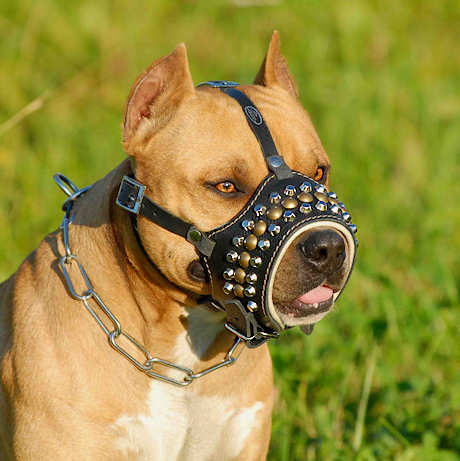This photograph, taken outdoors during the daytime, features a muscular, brown pit bull with a bit of white on its chest. The dog's ears are perked and clipped, and it gazes to the right from the lower left-hand corner of the square, three-by-three-inch image. The pit bull wears a distinctive black leather muzzle adorned with three rows of studs—gold in the center and silver on the outer rows. The muzzle is fastened with belt buckles under the ear and chin, leaving the dog's black nose and pink tongue visible. A wide chain-link choke collar encircles its neck. The background is a softly blurred expanse of green grass, suggesting the photo was taken in a field. The dog's intense, unfriendly gaze contributes to its formidable appearance.